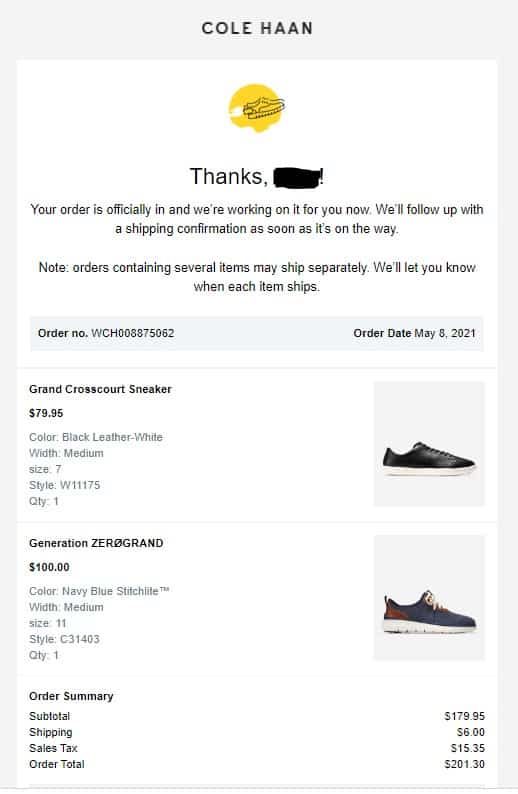Here is a detailed and cleaned-up caption for the given image:

---

This is a screenshot taken from either the Cole Haan app or the Cole Haan website, viewed on a smartphone. At the top of the screen, it prominently displays the Cole Haan logo: two hand-drawn shoes equipped with jet engines at the back, flying amidst some clouds inside a yellow circle, reminiscent of the sun.

Beneath the logo, there is a thank you message, followed by someone's name which has been blacked out with a sharpie. The message reads: "Your order is officially in and we're working on it now. We'll follow up with the shipping confirmation as soon as it's on its way." A note underneath specifies that orders containing several items may ship separately, and customers will be notified when each item ships.

On the left side of the screen, there is information regarding the order:
- Order number: WCH008875062
- Order date: May 8, 2021

The ordered items are listed below:
1. Grand Crosscourt Sneaker priced at $79.95
   - Color: Black Leather/White
   - Size: Medium 7
   - Style: W11175
   - Quantity: 1
   - An image of a sleek low-top sneaker with a white base and black leather upper is displayed to the right.
   
2. Generation ZERØGRAND priced at $100
   - Color: Navy Blue
   - Size: Medium 11
   - Style: C31403
   - Quantity: 1
   - An image of this shoe shows a stylish, athletic design ideal for running.

At the bottom of the screen, the order summary is listed:
- Subtotal: $179.95
- Shipping: $15.35
- Sales Tax: [assuming standard tax rate]
- Total: $195.30

---

This detailed caption carefully organizes and describes the content from the screenshot for clarity.